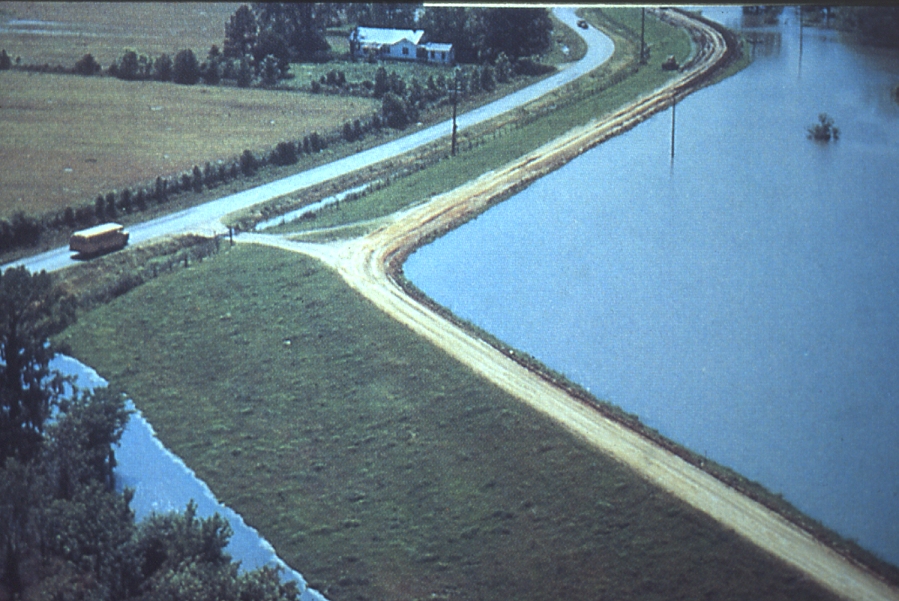This aerial daylight photograph captures a flood-affected rural landscape. A winding road cuts through the image, running parallel to an L-shaped, clear blue pond, which appears man-made. A yellow school bus is seen navigating this road, positioned in the bottom left corner, heading upward and curving left. To the left of the road lies a field and patches of grass. Scattered along the roadside are poles, some partially submerged in water, suggesting the area is possibly dealing with floodwaters. A prominent white, one-story house with a gabled roof stands near the top of the image, encircled by trees. Adjacent to this house are fields segmented by lines of trees. The flooded region extends to the right of the road, with visible submerged objects, implying a flood control levee in place, topped with a dirt path. This setting emphasizes a tranquil yet evidently flood-impacted rural scene.